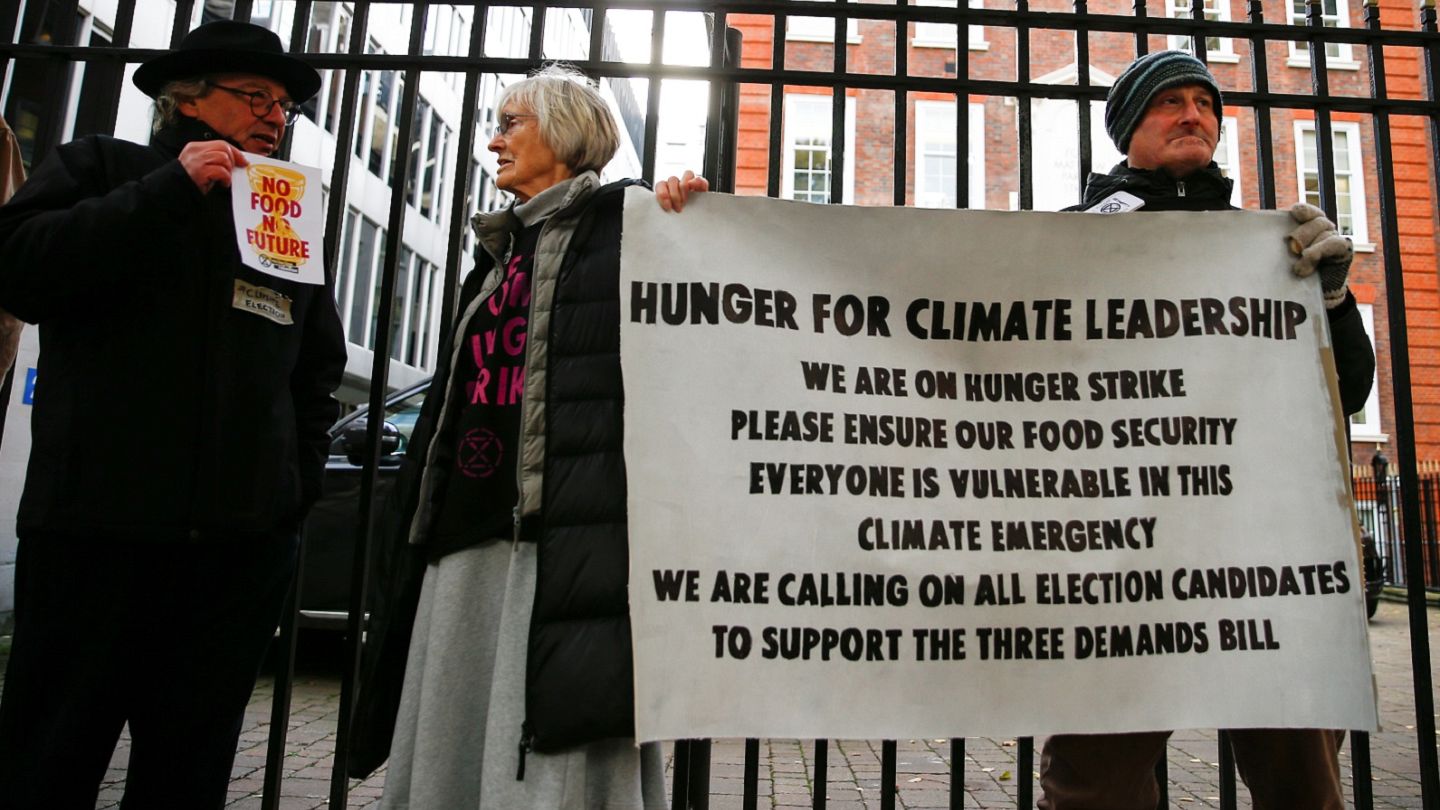The photo features three older Caucasian individuals engaged in a protest, positioned in front of a black gated fence with a large red-paneled or red-brick building looming behind them. On the left stands a man dressed in a black hat and black jacket, holding a sign with a golden chalice and red text that reads "No Food, No Future." To his right, a woman wearing a black puffer jacket over a gray dress or skirt, and glasses, faces him while jointly holding a large white banner with another man. This man, on the far right, is also older, donning a gray beanie and gloves. Both the woman and the man hold up a sign with black text stating, "Hunger for Climate Leadership. We are on hunger strike. Please ensure our food security. Everyone is vulnerable in this climate emergency. We are calling on all election candidates to support the Three Demands Bill." The setting is completed with additional white buildings visible to the left behind the black fence.